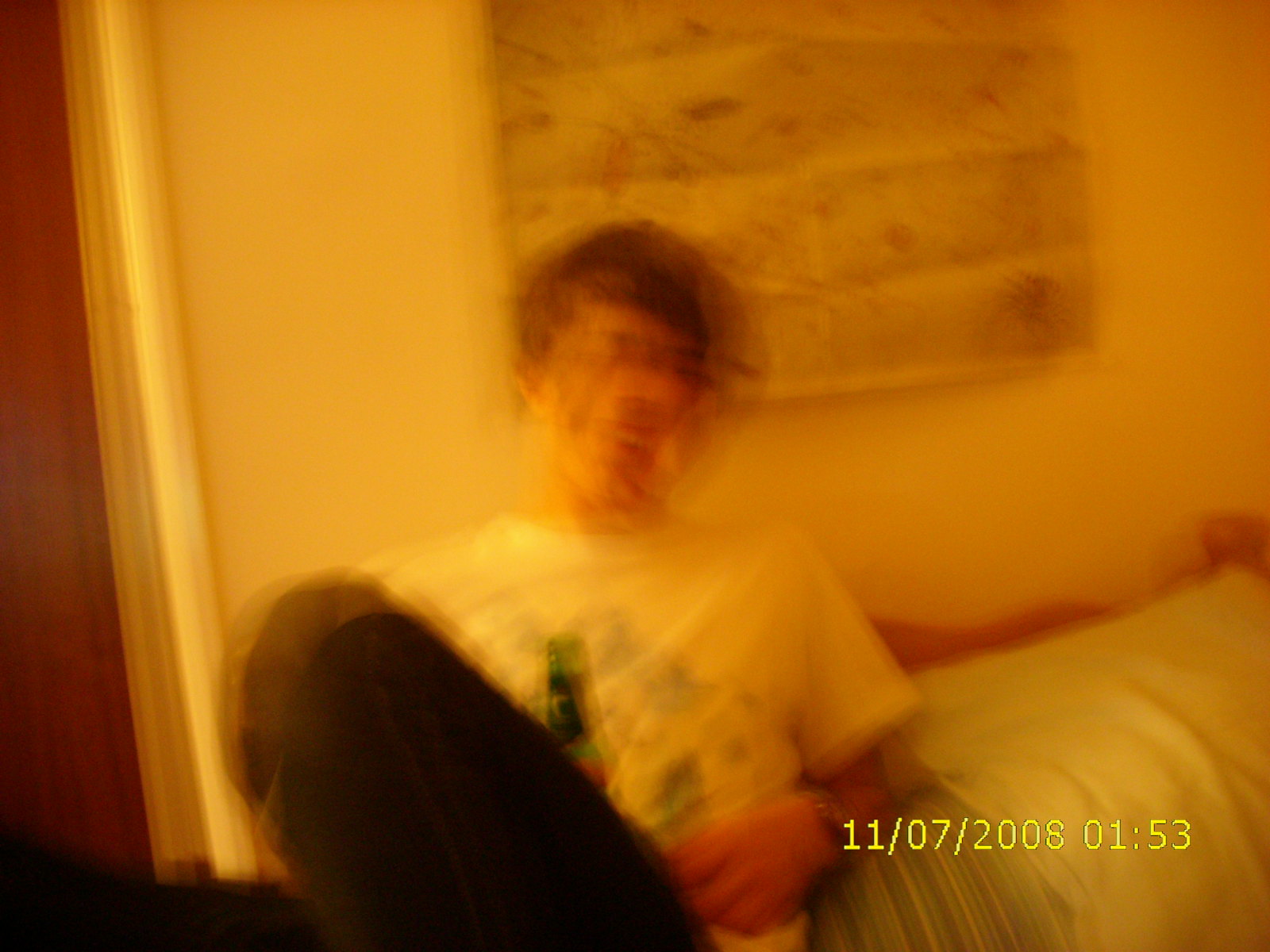This image captures a blurry and out-of-focus depiction of a young man with short, dark hair, appearing to smile or laugh. The entire image is washed with a yellowish or golden tint, suggesting it was taken in movement. The timestamp "11-07-2008-01:53" is prominently displayed in yellow at the bottom right corner. The individual, who has a light skin tone, wears a white t-shirt adorned with some sort of graphic and black jeans. He's in a seated position, possibly against a bed or a similar sitting surface, with one knee up and a green beer bottle held near his chest. His mouth appears open, showing his teeth, and he may be wearing a wristwatch. The setting features white walls with some indistinct wall art or covering in the background. The overall blur of the image obscures finer details, emphasizing the motion and ambient light conditions at the time the photo was taken.